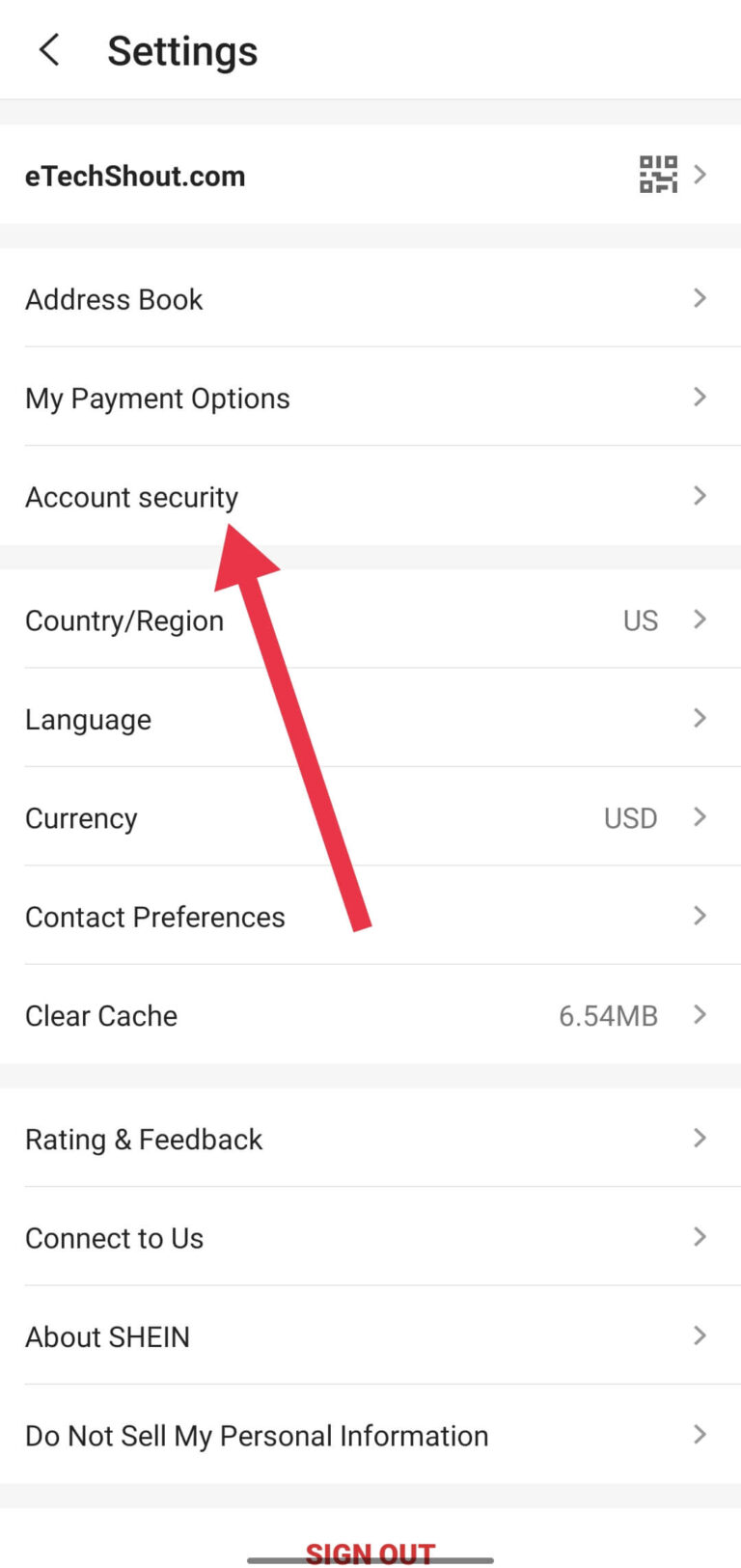A screenshot of a phone displays the "Settings" menu. At the top, a back arrow and the word "Settings" are visible, followed by a pale gray line. Below it, "etechshout.com" and a QR code are presented, separated by another gray line. The menu items listed include "Address Book," "My Payment Options," and "Account Security," which is highlighted with a prominent red arrow. Further down, under another gray line, the settings continue with "Country/Region: US," "Language," "Currency: USD," "Contact Preferences," and "Clear Cache (6.54 MB)." Another pale gray line follows before the options "Rating and Feedback," "Contact Us," "About Shein," and "Do Not Sell My Personal Information." The menu culminates with a gray line and the "Sign Out" option in bold red capital letters at the bottom.